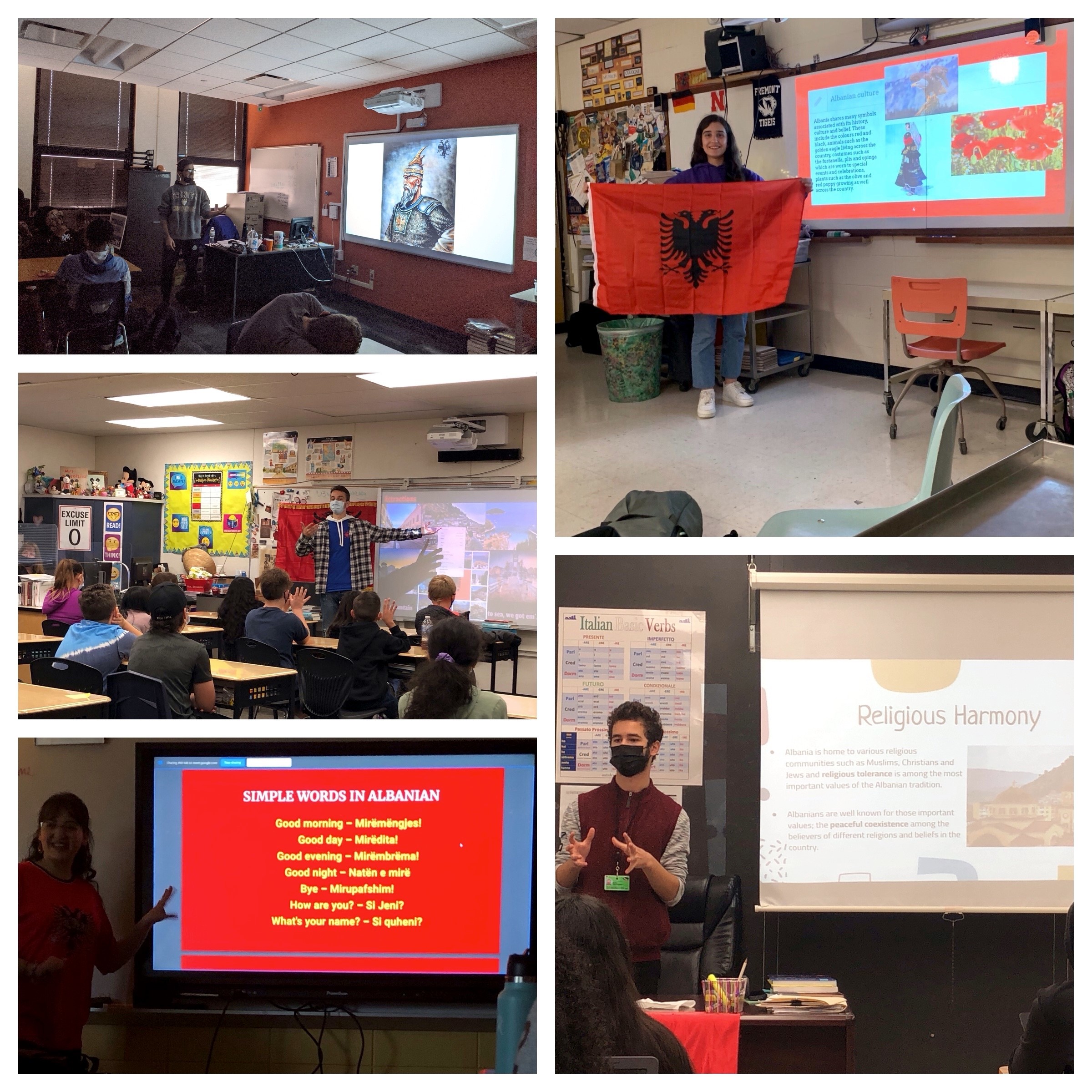This is a collection of five images depicting different classroom settings where presentations are being given. The top image shows a classroom with a red wall and a projector screen displaying a medieval painting. In the second picture, a teacher in a plaid jacket and wearing a face mask points at a projector screen that says "Religious Harmony." The third picture features another teacher pointing at a projector screen with the phrase "Simple words in Albanian." The fourth image captures a teacher holding up a red flag with an image on it while standing in front of a projector screen. The fifth picture shows yet another teacher, wearing a black face mask, gesturing towards the class while a projected image is displayed.